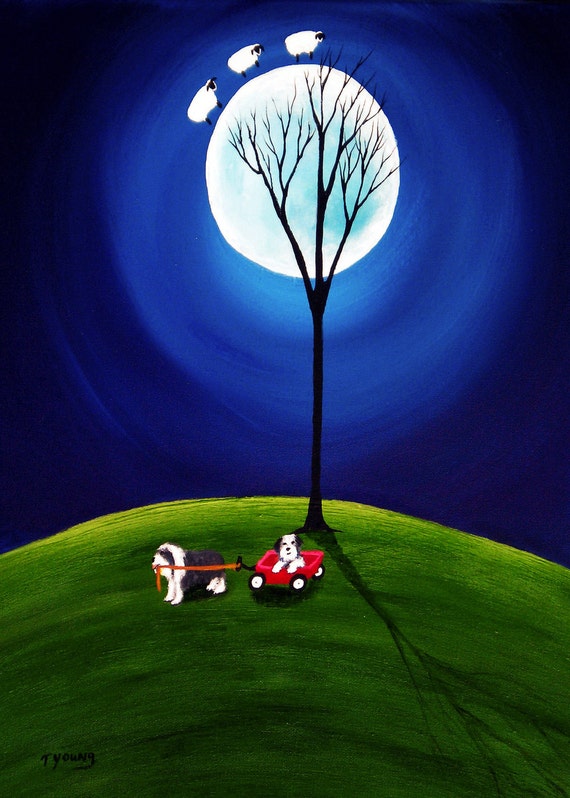This illustration, possibly crafted as an oil on canvas or perhaps computer-generated, is signed by T. Young in the bottom left corner. It portrays a serene nighttime scene set against a dark blue sky. The focal point is a St. Bernard-like dog with long black and white fur, gripping a rope in its mouth to pull a red wagon. Seated in the wagon is a smaller dog, possibly a puppy, suggesting a familial bond between the two. They traverse a plush, green hill, adorned with a bare tree that stretches upwards, casting moonlit shadows and partially obscuring the glowing moon. Adding a whimsical touch, three sheep appear to frolic atop the illuminating sphere in the sky.